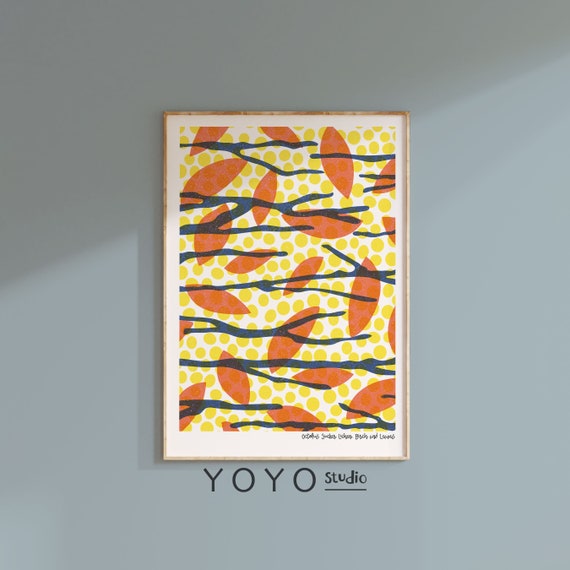The artwork is a framed print encased in a thin, light-colored frame with a white border surrounding the print. It features a pattern of medium-sized yellow polka dots as the background, with gray and blue branches splayed across. Superimposed on these branches are numerous orange, football-shaped leaves that appear to be falling throughout the print. The art is titled with the text "Yo-Yo Studio" inscribed below. This print is displayed on a wall that is predominantly gray, with shades varying from light to dark gray, and serves as a focal point in the space. Additionally, there's a small blue text at the bottom of the print.